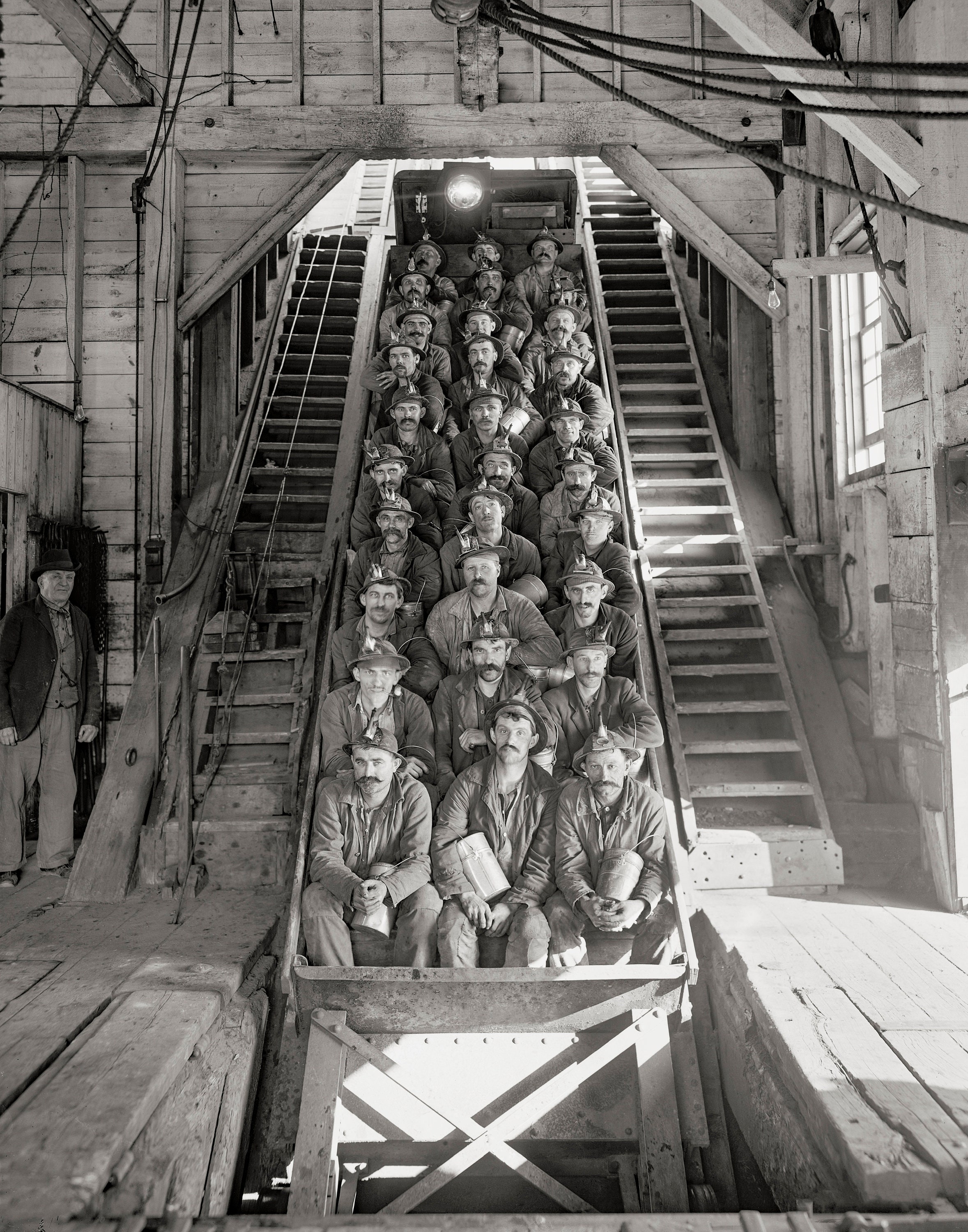This is a detailed black-and-white photograph capturing a group of approximately 30 mine workers seated in an old wooden mine cart designed to carry them down into the depths of a mine. The cart, angled at about 45 degrees ready for descent, is arranged with ten rows of three men each, although one row has only two individuals. Each miner is equipped with a helmet—some adorned with lights or unidentifiable attachments—and they are all holding metal buckets, likely for their lunch or mining work. The cart is flanked by steep wooden staircases on either side, allowing access to the platform. A single, large light bulb hangs above the cart to illuminate their way down. To the far left stands an older man in a suit, coat, and top hat, possibly the mine owner or operator of the cart; he appears distinct from the miners, who are dressed in work attire, including hats and jeans. The interior of the mine shaft, entirely constructed from wood, also features overhead cables running from the top to the top right of the image. Many of the miners are smiling at the camera, adding a human touch to this historical snapshot of early industrial labor.